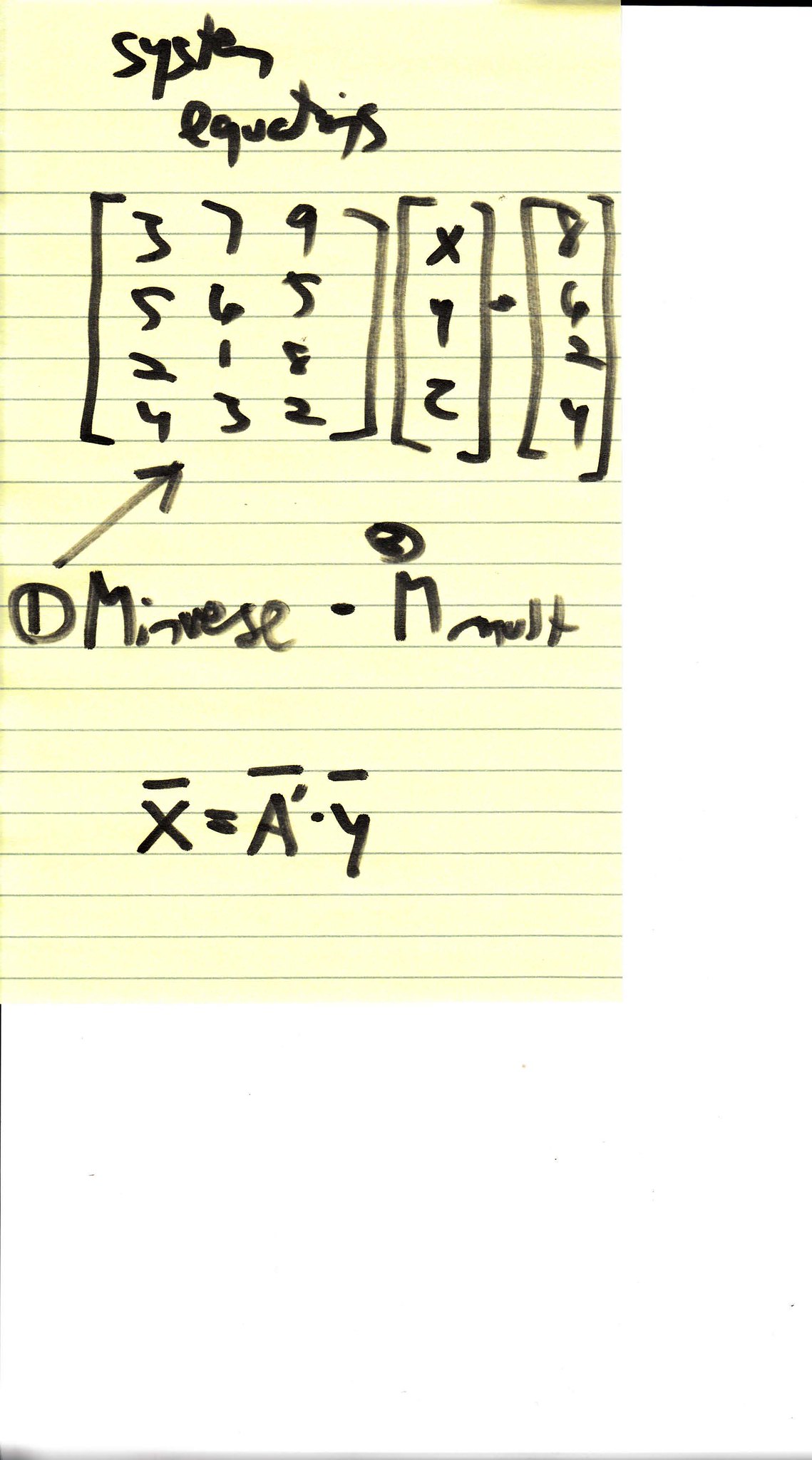This is a hand-drawn sketch of a complex mathematical equation, rendered with a black marker on a yellowish or white piece of lined paper. The writing is somewhat messy, and the paper appears to have been scanned or photocopied, as evidenced by the background’s white space with a black vertical line and a section of blackish-gray material at the bottom.

The focal point of the image is a large bracket enclosing three columns of numbers: 
- The first column contains the numbers 3, 5, 2, and 4.
- The second column lists the numbers 7, 6, 1, and 3.
- The third column includes the numbers 9, 5, 8, and 2.

Next to this bracketed array of numbers is another open bracket containing the variables X, Y, and Z. Following this is a closed bracket, and then a dot signifying multiplication. There is another bracket with a single column of numbers 8, 6, 2, and 4 enclosed within it.

Additionally, a circled number 1 points towards the initial arrangement of three columns of numbers, and next to it are the expressions “M inverse” and “M mult”, with “M inverse” suggesting the matrix inverse of M, and “M mult” indicating multiplication by M. This gives the impression of an equation representing the inverse of M minus M multiplied by a vector consisting of X, Y, Z, and the numbers 8, 6, 2, 4.

Below this complex bracketed expression, another line reads: 
\[ \bar{X} = A' \cdot \bar{Y} \]
Here, \(\bar{X}\) represents a variable X with a bar over it, and \(A'\) signifies a capital A with an apostrophe, followed by a dot implying multiplication with \(\bar{Y}\), a variable Y with a bar over it.

In summary, the sketch presents an intricate mathematical setup involving matrices, inverse operations, and multiplication, all depicted on a lined piece of paper with a somewhat cluttered and hand-drawn appearance.